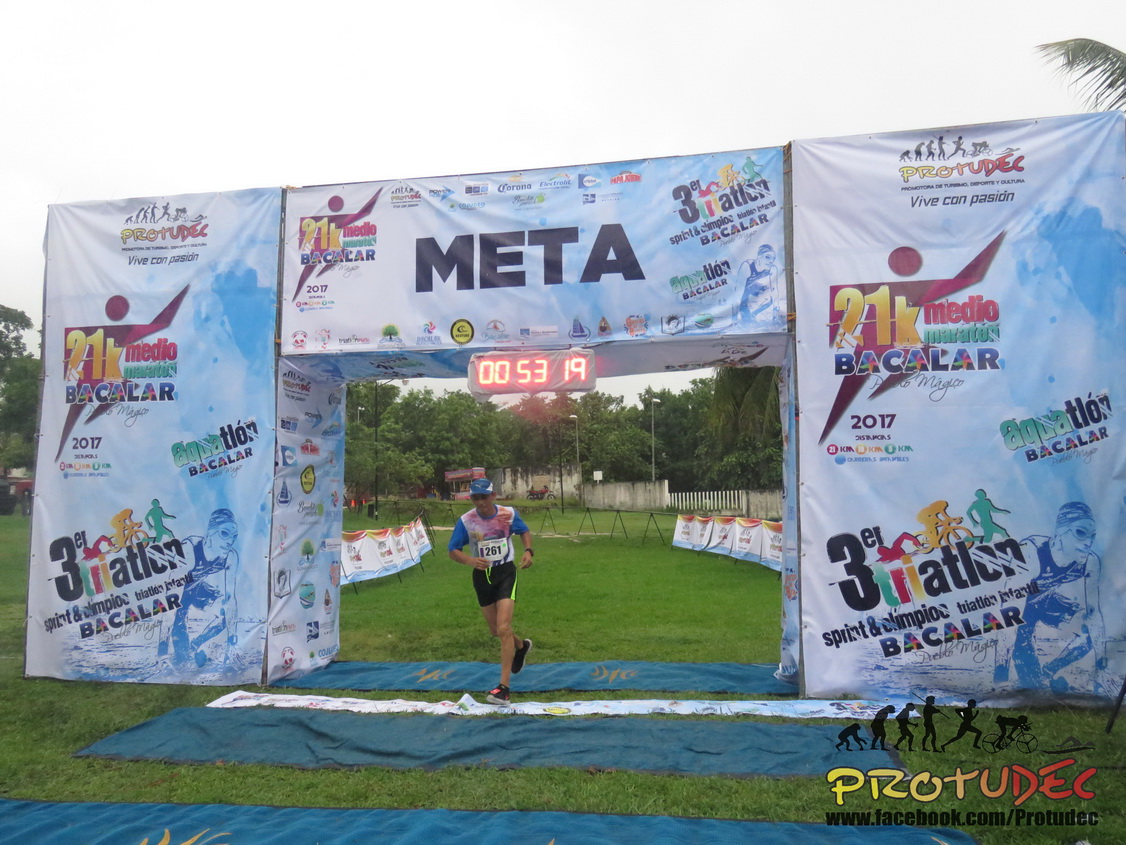A detailed image shows a finish line setup for a triathlon, featuring an archway structure adorned with various event and sponsor signage. At the center and top of the arch, the word “META” is prominently displayed, potentially indicating a sponsorship. The arch itself resembles a rectangular frame with a gap at the bottom for participants to pass through. Beneath this gap, a digital timer reads 00:53:19, signifying a recorded time.

The arch is festooned with multiple event logos and inscriptions, although some may be difficult to discern due to the image quality. Clearly visible are the phrases "21K Medio Marathon Bacalar," "3ER Triathlon," and "Sprint and Olympio." Additional sponsor names and images of sports icons further decorate the structure. The race appears to be taking place in an area surrounded by trees, contributing to the overall lively and open environment of the event.

Positioned directly below the timer, an athlete, identified as contestant number 261, is captured mid-stride. He is donned in black shorts, a blue shirt, a blue cap, and black shoes, clearly engaged in the intense competition, embodying the spirit of the triathlon. The image also includes a watermark at the bottom reading “PROTUDEC,” with the accompanying link "facebook.com/protudec."